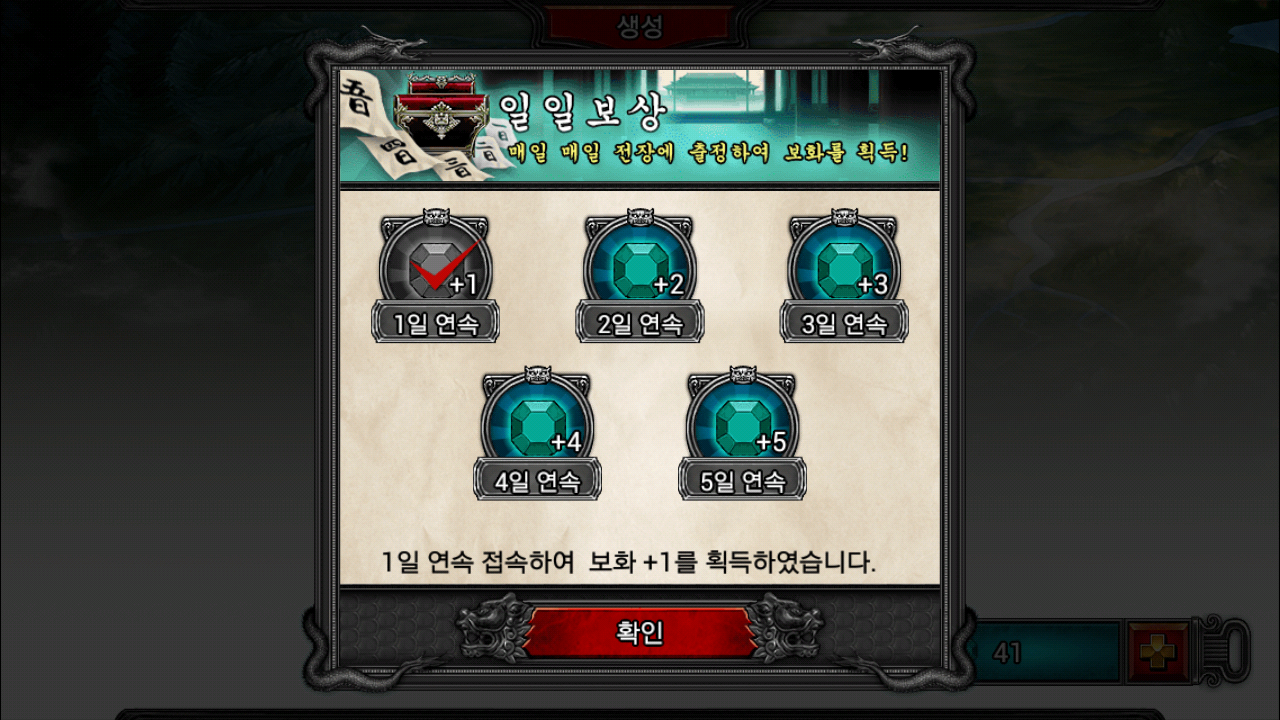The image is a detailed screenshot from a Korean mobile video game. The background transitions from deep black at the top to dark gray at the bottom. Central to the image is an ornate pop-up box, bordered with a decorative frame featuring dragon heads with their mouths open at all four corners. Within this framed box are five gem designs. The gem in the top left is grayed out with a check mark, indicating it has been acquired, while the other four gems are still in color, labeled with numbers. At the bottom center of the pop-up box, a red button adorned with dragon heads flanks either side. The background outside the box resembles dark, stormy clouds, adding to the dramatic atmosphere.